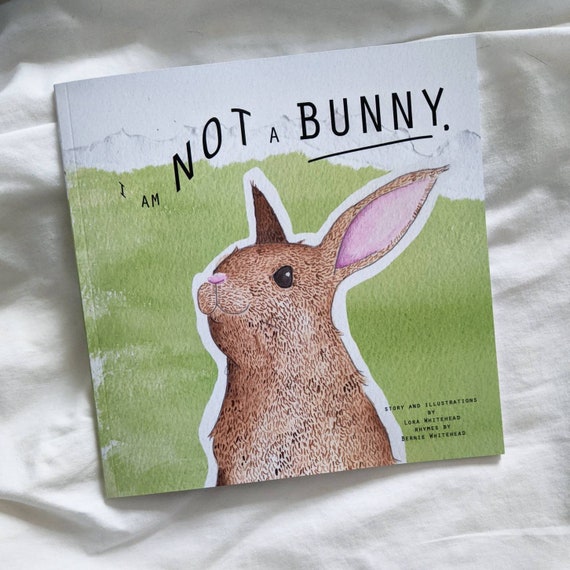The image depicts the front cover of a thin, hardcover children's book titled "I Am NOT a Bunny," laying on a cotton white sheet background. The book cover features a predominantly white upper section resembling mountains under a white sky, while the lower portion showcases a light green grassy field. Centrally positioned in this grassy area is a close-up, hand-illustrated rabbit. The rabbit, with fluffy brown fur, stands on its hind legs and gazes directly at the viewer with its expressive black eyes. It has a pink nose, pink insides of its ears, and a slight smile. The title, "I Am NOT a Bunny," is written in black font with the words "NOT" and "bunny" emphasized in larger font, arranged in a somewhat wavy pattern. The bottom right corner of the cover includes the credits: "Story and illustrations by Laura Whitehead, rhymes by Bernie Whitehead." This charming bunny looks directly at you, potentially intriguing viewers to pick up the book.